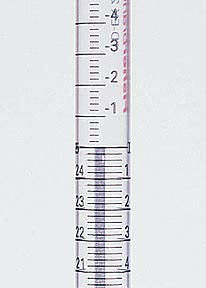A detailed image in portrait format showcases a glass measuring device, possibly a thermometer or a chemist's measuring tube, set against a uniform grey background. The slender, transparent tube extends vertically from the top centre to the bottom centre of the image. 

Beginning at the lower portion of the tube, the left side is marked with ascending numbers: 21, 22, 23, and 24, each accompanied by precise calibration lines. The right side of this segment features descending numbers: 4, 3, 2, and 1, similarly interspersed with calibration marks.

Moving upwards, the tube undergoes a distinct transformation. The calibration system changes, with central markings displaying consecutive negative numbers: -1, -2, -3, -4, and the digit 4. Unlike the lower half, this segment lacks numerical markings on either side. The top portion also features red lettering, likely indicating the maker or brand, though its exact inscription remains obscured, possibly due to its positioning on the interior or reverse side of the tube.

The contrasting calibration methods and enigmatic red inscription give the impression of two images superimposed or a uniquely designed measuring instrument. This sophisticated glass tube, configured for precision measurement, is a typical tool you might encounter in a chemistry laboratory.